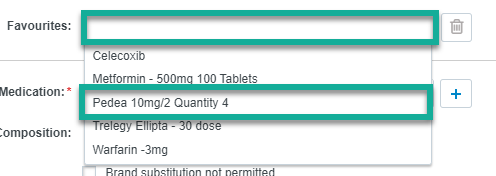This horizontal, left-to-right image appears to be a screenshot or screen grab from a computer or smart device. The background is primarily a plain white, derived from the screen itself.

Left-aligned along the image, we can see several bolded sections:
- **Favorites**: Displayed in bold black text, followed by a white empty box with a green border that lists "Cellococcib or Metformin, 500 milligrams, 100 tablets." A trash can icon is visible to the right of this entry.
- **Medication**: A bold black heading with a star next to it, denoting importance. This section includes a green-bordered box that reads "Pedia, 10 milligrams / Quantity: 4."
- **Composition**: This section lists "Trilogy, Alipita, 30 dose, Warfarin, 3 milligrams," with an unchecked box that states "Brand substitution not permitted."

On the far right beneath the trash can icon, there's another small box featuring a blue plus sign.